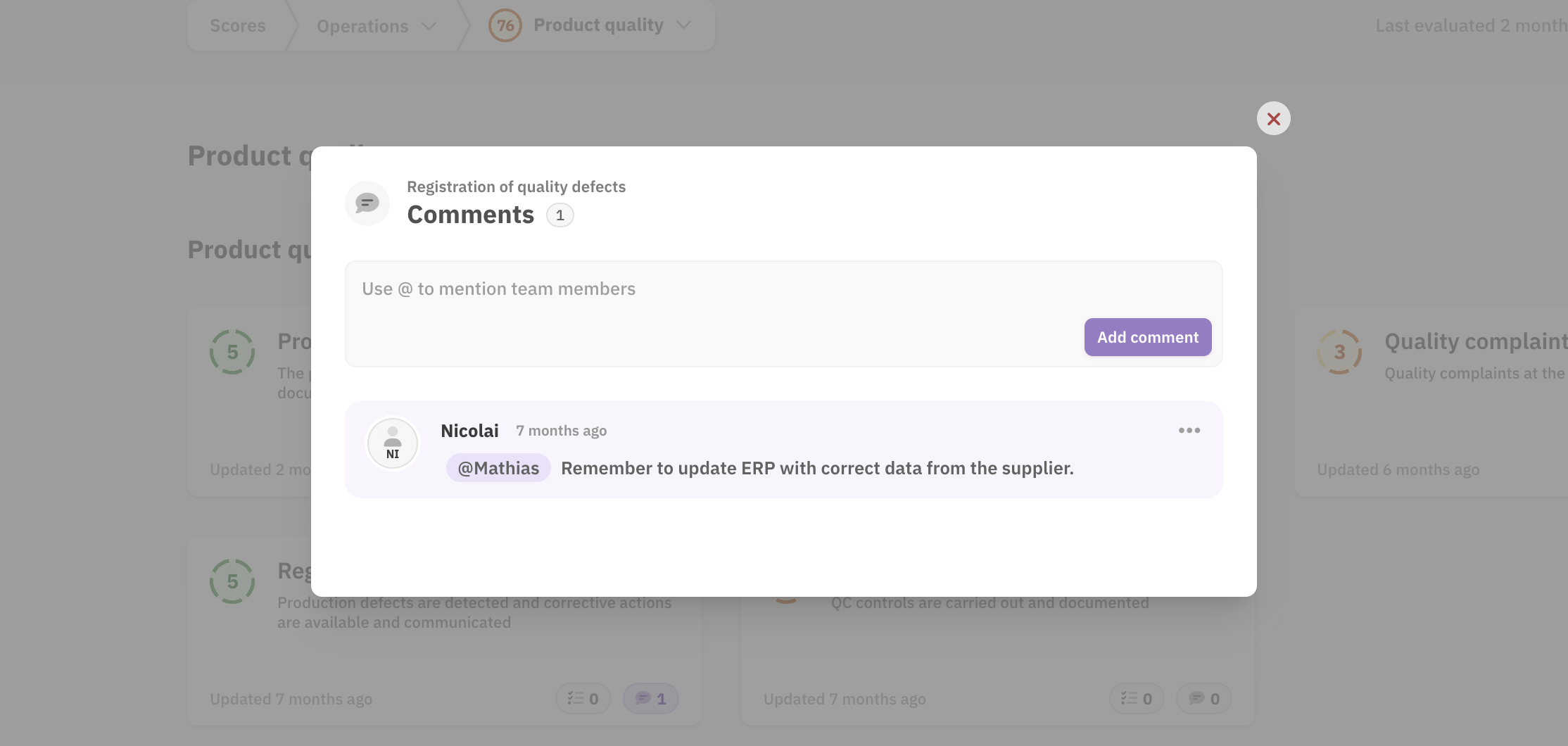In this image, we can see a detailed view of a product feedback and registration section. At the top of the image, the headings "Scores Operations" and "Product Quality" are visible. Under "Product Quality," a numerical score of 76 is displayed. Below this, there are ratings indicated with numbers in different colors; green numbers denote ratings of five, while an orange-colored rating of three is displayed to the right.

Additionally, there is a white pop-up screen featuring a section titled "Registration of Quality Defects Comments." This section includes a text box with a placeholder message instructing users to "use @ to mention team members." At the bottom right of this pop-up screen, there is an "Add Comment" button.

Below this, a historical comment from a user named Nikolai, posted seven months ago, is visible. The comment reads, “Matthias, remember to update ERP with correct data from the supplier.”